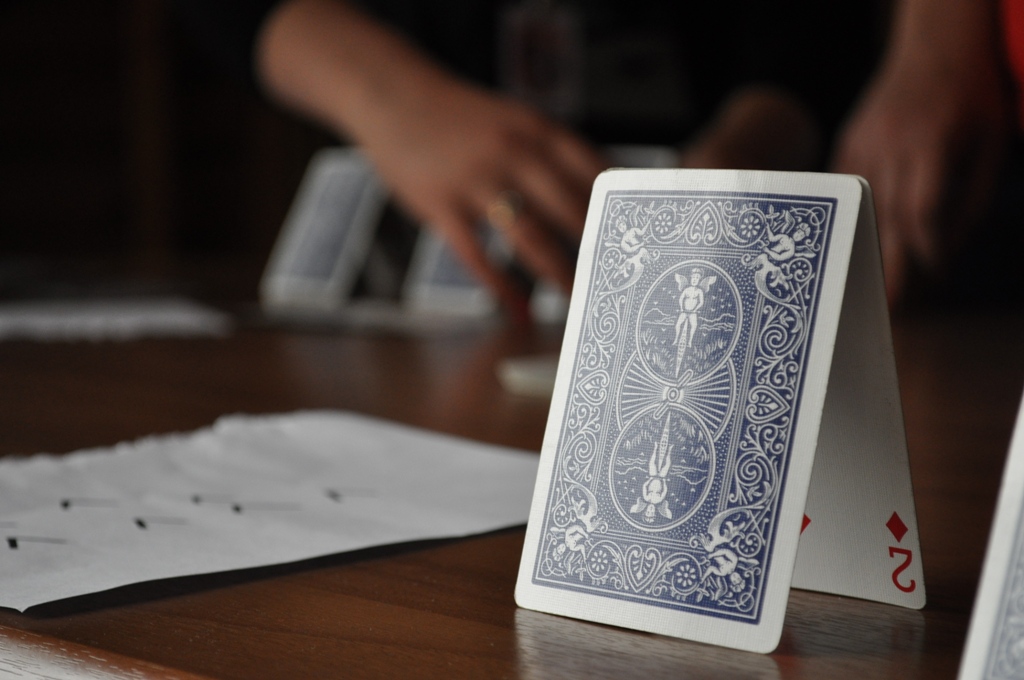This detailed close-up captures the nascent stages of a card tower. The central focus is on two cards meticulously angled against each other, forming a delicate triangular structure without a base. The viewer can observe the back of one card, which features the classic Bicycle playing card design in blue, adorned with cherubs riding bicycles at the top and bottom and surrounded by an ornate border. The adjacent card's face, a two of hearts, is prominently visible, adding a splash of white and red to the scene.

The cards are resting on a refined dark wooden table, enhancing the contrast and highlighting the intricate details of the cards. To the left, slightly out of focus, lies a white piece of paper speckled with colorful dots, subtly adding an element of curiosity. In the distant background, blurred by depth of field, a man's hands are visible, seemingly engaged in the act of picking up another object, likely to further the construction of the card tower. This glimpse into the meticulous process adds a dynamic element to the otherwise static scene.